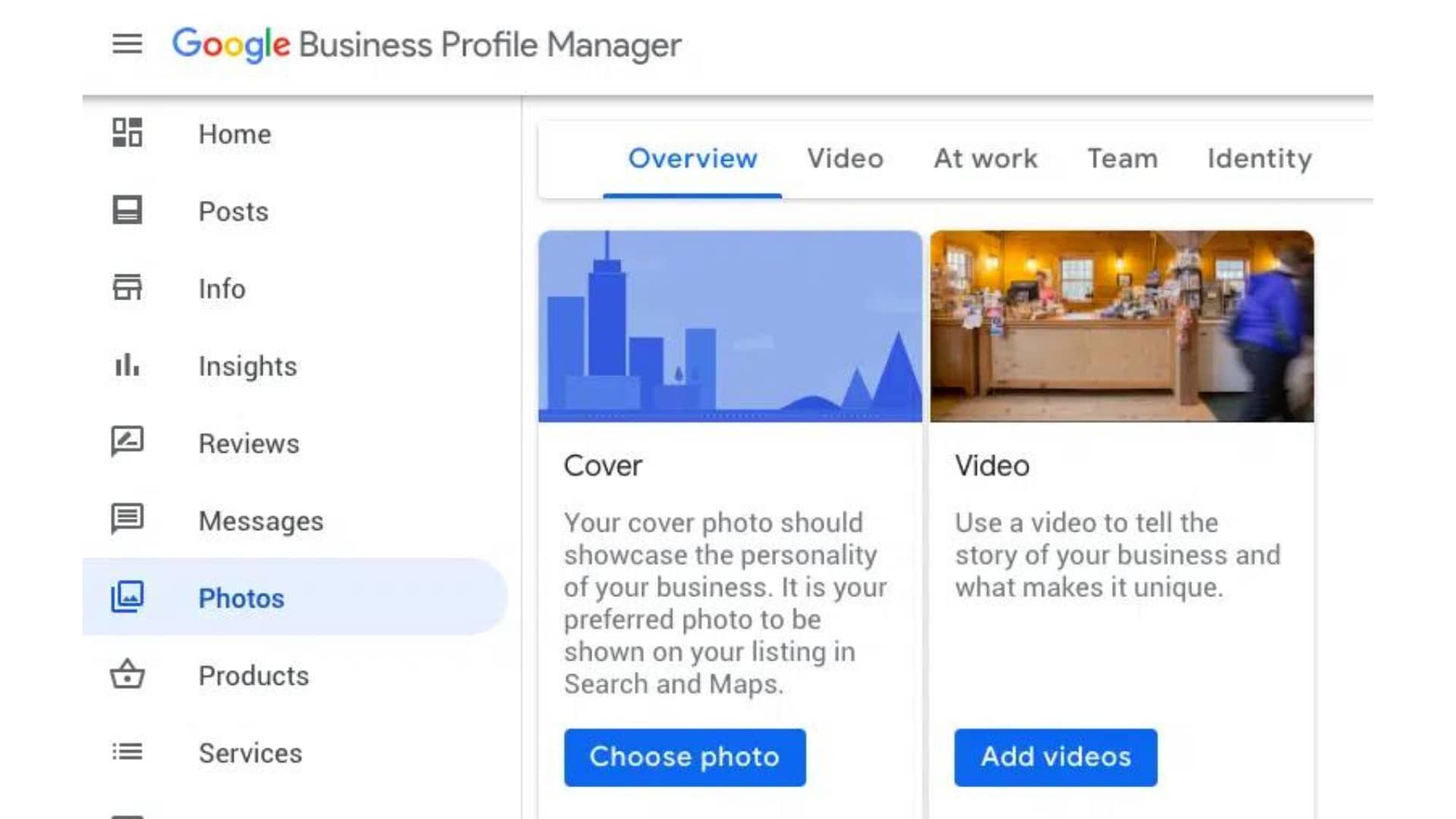This image is a screenshot from the Google Business Profile Manager web application. At the top, the interface prominently displays the Google logo in its iconic colors of blue, red, yellow, and green, followed by the text "Business Profile Manager." To the left of these title elements, there is a three-line hamburger menu button.

On the left side of the screen, a vertical navigation menu lists various sections of the Google Business Profile Manager, such as Home, Posts, Info, Insights, Reviews, Messages, Photos, Products, and Services. These options are presented sequentially, each accompanied by a representative icon. Currently, the "Photos" section is selected, as indicated by its light blue highlight, contrasting against the default black text on a white background of the unselected options.

The right side of the screen displays the contents of the "Photos" section, subdivided into five categories at the top: Overview, Video, At Work, Team, and Identity. The "Overview" category is currently selected, revealing two subsections underneath: "Cover" and "Video." Users are given the option to either choose a photo by clicking a blue button labeled "Choose a photo" or add a video by clicking a similarly styled blue button labeled "Add a video."